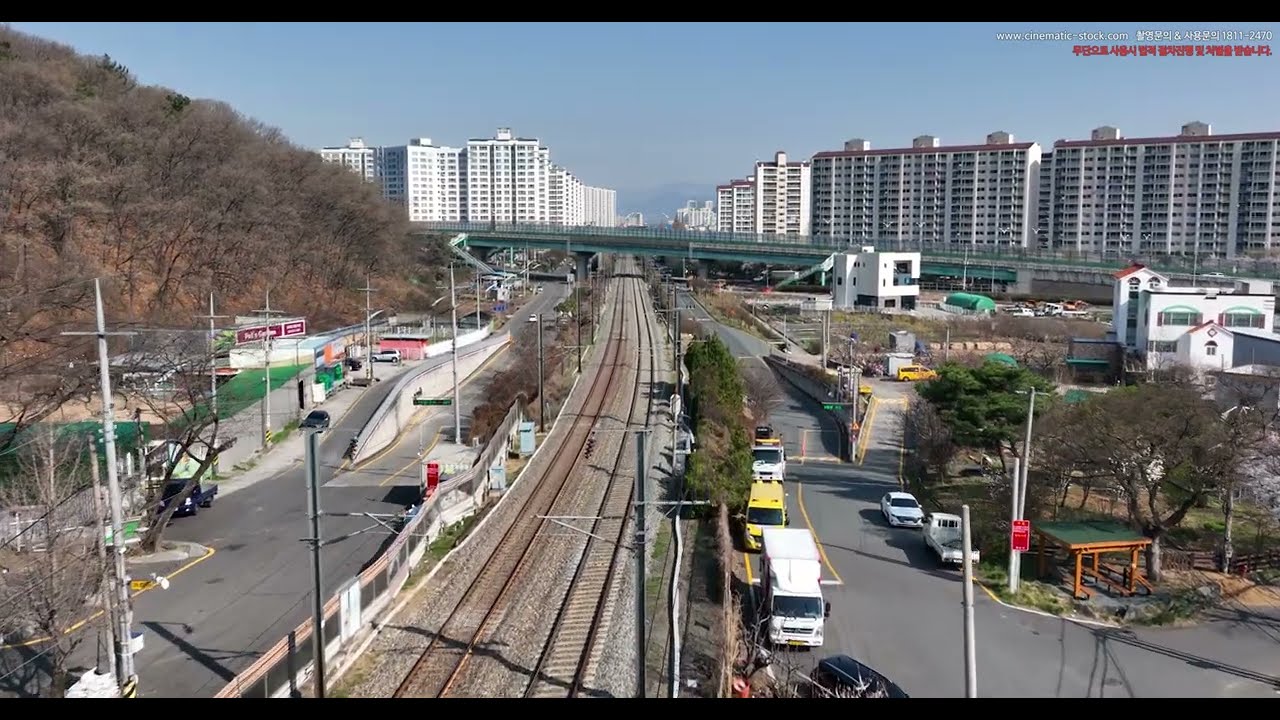This aerial photograph, likely taken from a drone, bridge, or a building around three or four stories high, captures a high-angle view of a cityscape intersected by a pair of railroad tracks running directly ahead and tapering into the horizon. The area exhibits a rundown, industrial aesthetic with various businesses, trucks, and cars scattered along the paved streets. On the left, a small hill with sparse trees suggests a seasonal setting, potentially winter. The right side of the image features a mix of residential and industrial elements, including older buildings and an apartment complex. In the distance, several very tall, uniform apartment complexes, each approximately 15-20 stories high, dominate the skyline. These buildings, with flat roofs and additional small structures on top, suggest an urbanized landscape, possibly in an Eastern European country due to the style of vehicles and construction. Despite the industrial feel, some greenery and vegetation are present, offering a contrast to the otherwise aged surroundings.